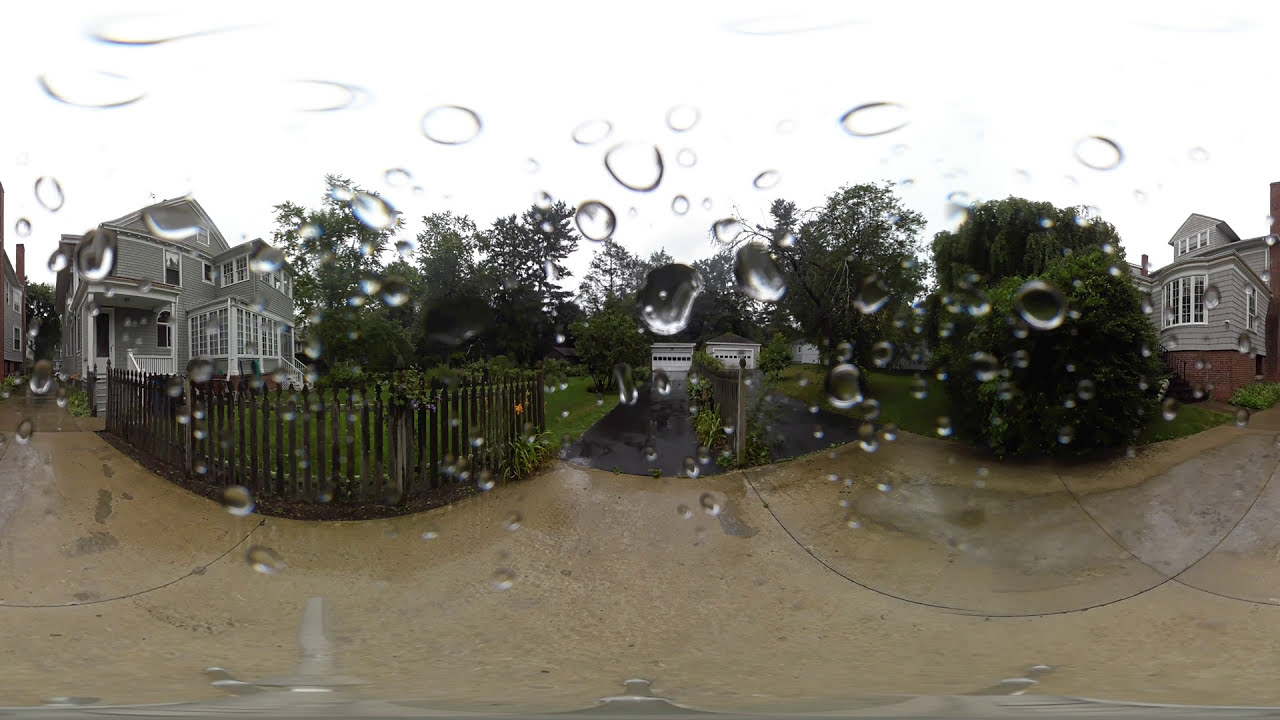A striking fisheye lens capture of a neighborhood scene on a rainy day. The image prominently features two gray houses with white trim on opposite sides of the scene—one on the far left with flat porch panels and white-railed windows, and one on the far right with a distinct rounded attic window with three panels. Drops of water cover the camera lens, blurring the view and adding a textured layer of distortion. Between the two homes are garages with white doors, differentiated by the size of their top windows. A weathered, brown picket fence spans in front of the house on the left, and both houses are connected by a black asphalt driveway that is visibly drenched from the rain. The ground appears saturated, with a yellowish tint that might suggest waterlogged dirt. In the far background, lush dark green trees full of leaves rise against an overcast, nearly white sky, emphasizing the hazy and overcast atmosphere of this rainy day.